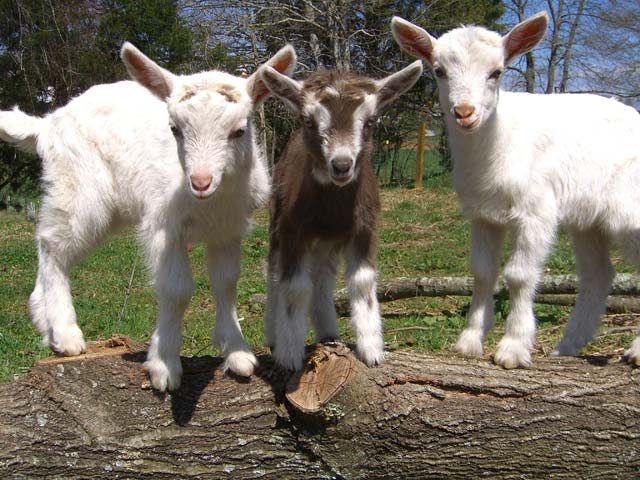In this picturesque image, three adorable baby goats, likely less than a year old, are showcased. Two of the goats, positioned on the left and right, are pure white, while the one in the middle sports a distinctive blend of dark brown and white, with white fur resembling stockings on its legs. All three goats are cutely peering straight into the camera, giving the impression of a staged photo shoot. They are standing with their front paws on a substantial log, possibly from a fallen tree, which spans the bottom of the photograph and features a notable knot. The background is a mix of lush, unkempt green grass and twisting trees, some bare and others adorned with green leaves, against a clear blue sky. The goats' ears are perked up at high angles, showing the pink insides, adding to their friendly and endearing appearance. A stick is also visible just behind the trio.